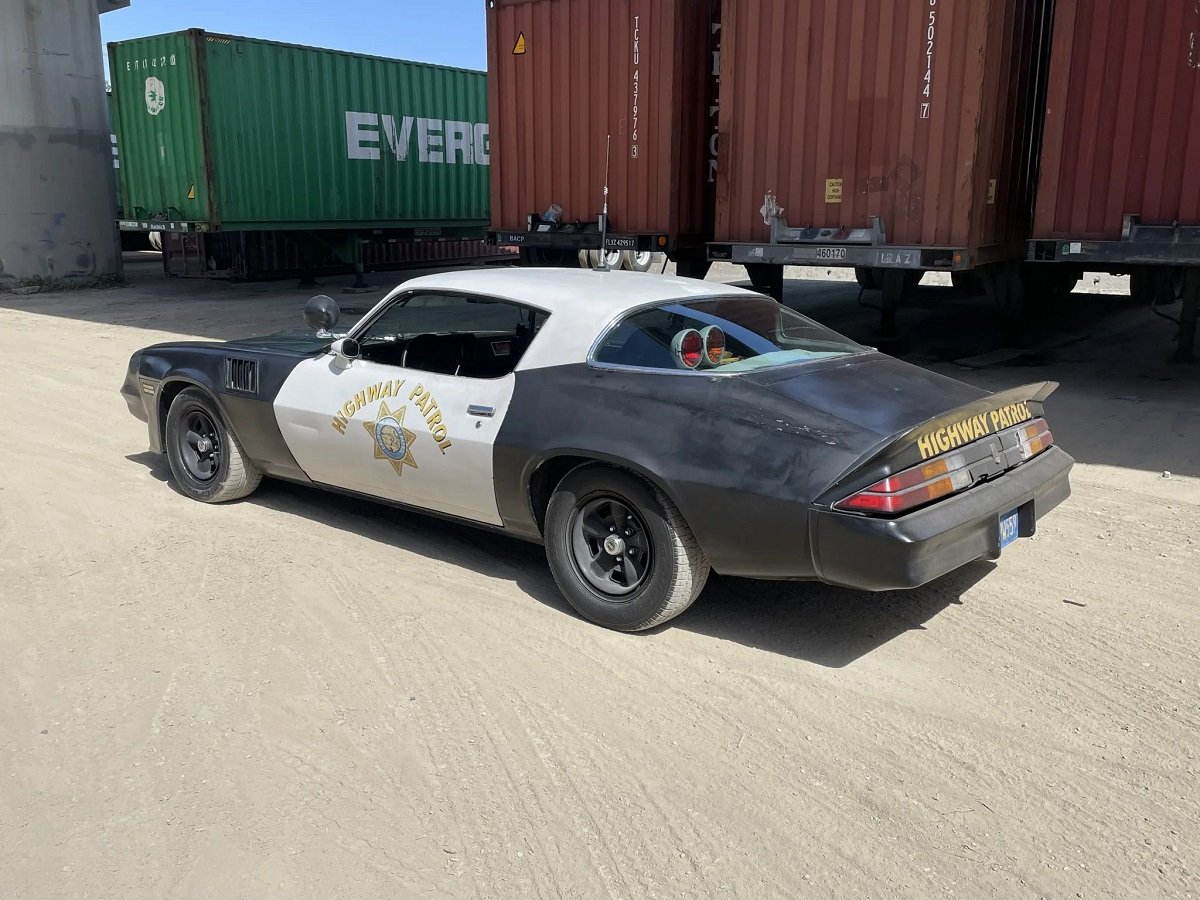The image depicts an outdoor parking lot filled with several large trucks and a dusty highway patrol car. On the upper left section of the image, there's a large concrete cylinder positioned adjacent to a green truck marked with the partially visible company name "Evergreen," the letters "E-V-E-R-G" printed in white. Moving rightward, there are three maroon red trucks parked side by side, and their backs can be seen clearly.

In front of these trucks, there is a black and white highway patrol car, primarily black with a white band running from the driver's side door over the roof and to the other side. It features the text "Highway Patrol" in yellow, along with a gold star badge that has a blue circular logo in the center. This star and text are prominently displayed on the side and towards the end of the car. The car’s license plate is blue, though the specific details are unclear. The patrol car is situated on a gray dirt area, and above the car, several shipping containers are visible, with the green one on the far left and the three maroon red ones to its right.